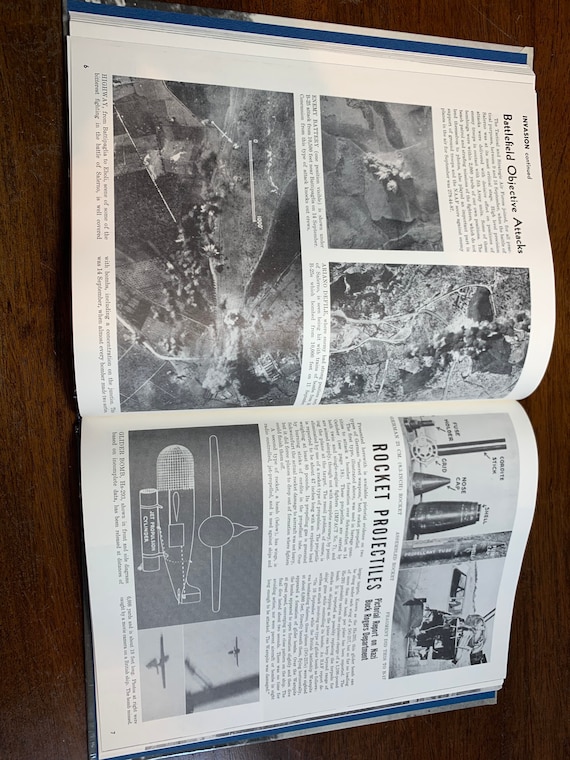This photograph features an open book placed on a brown wooden table, oriented vertically and requiring a counterclockwise rotation to read properly. The book appears to be a larger format, akin to a picture book but intended for adults. Its pages are monochrome, filled with a blend of text and images. 

On the left page, which is labeled "Battlefield Objective Attacks" at the top in bold black letters, there are aerial photographs depicting areas under bombardment, showing clouds of smoke rising from the ground below. On the right page, labeled "Rocket Projectiles," there are detailed schematics of rockets and various aircraft components. Each page includes paragraphs that elaborate on the accompanying images and topics. The chapter or section appears to be titled "Invasion," and the book is currently open to pages six and seven.